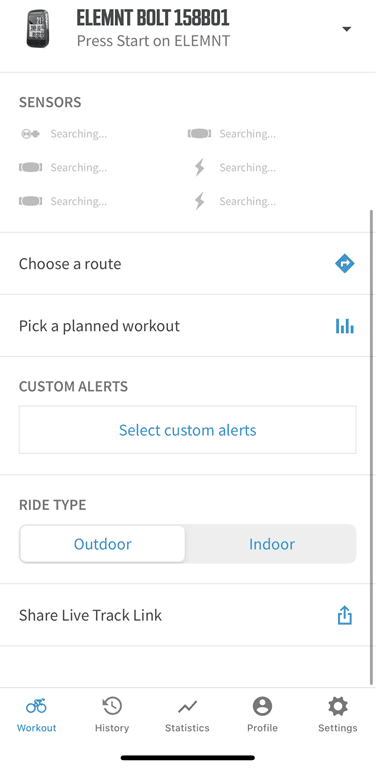This smartphone screenshot displays the interface of the ELEMNT Bolt 158B01 application web page. At the top, the ELEMNT logo is visible, resembling a smartphone. Beneath the logo, there is a "Press Start on ELEMNT" prompt accompanied by a drop-down arrow on the right. A light gray line marked "Sensors" follows, under which multiple vertically aligned "Searching" icons are visible. To the right side, additional "Searching" icons are displayed alongside lightning bolt symbols. This section is separated by another thin line labeled "Choose a Route," featuring a black triangle with a white right-facing arrow underneath. 

Continuing downward, another dividing line precedes the section "Pick a Planned Workout," characterized by graphical representations of alternating long and short horizontal lines. Following is the "Custom Alerts" section with a "Select Custom Alerts" button, segregated by another thin line. Subsequently, there's a "Ride Type" section with two buttons labeled "Outdoor" and "Indoor." Below this is the text "Share Live Track Link" paired with an Upload button. At the bottom of the screen, icons for "Workout," "History," "Statistics," "Profile," and "Settings" are presented, with a "Home" button situated at the very base.